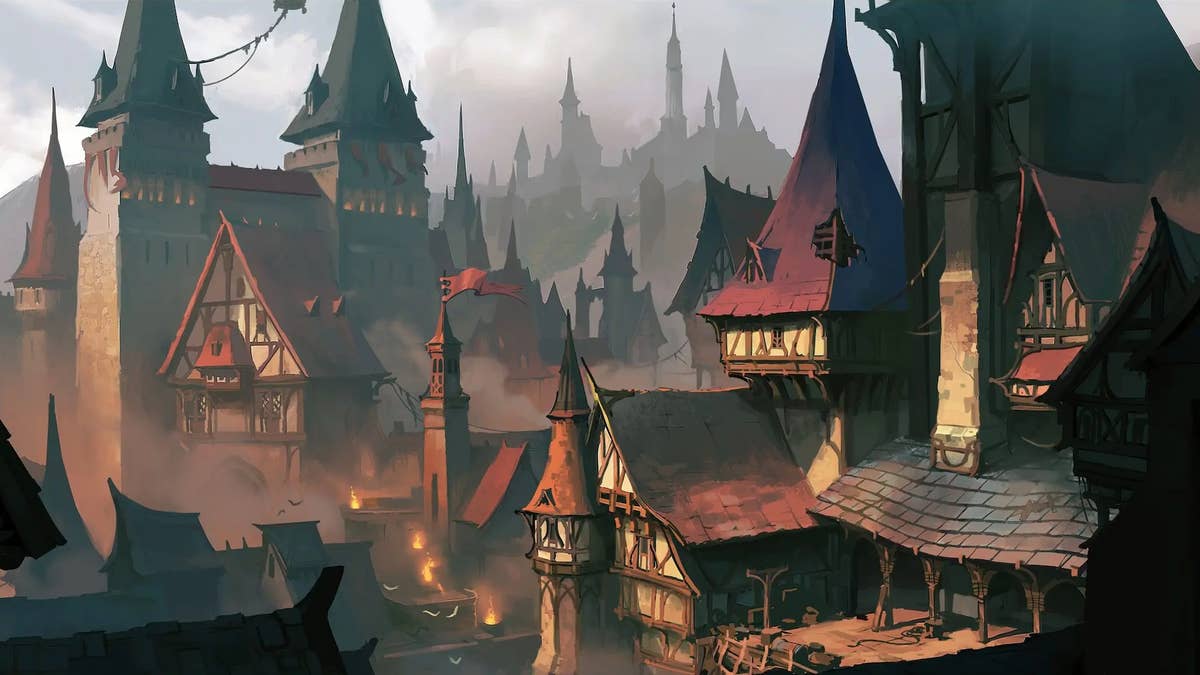This pixel art image, likely a frame from a video game, intricately depicts a medieval town under a gray, overcast sky. Dominated by rows of complex buildings featuring multiple wings, stories, and various levels of turrets, the scene exudes an old-world charm. The building on the left is roughly square, adorned with two corner towers and a smaller wing in front that faces sideways, all topped with gabled roofs. Most buildings exhibit Tudor-style half-timbers, complemented by slate or shingled roofs in shades of red and gray. The image's color palette employs mostly black and white, light brown, and red hues. In the foreground to the left, a fire burns in kettles, adding an element of warmth and rustic activity to the scene. A red flag adorns one of the structures. The castle silhouette and a row of towered buildings stretch across the horizon, while sunlight pierces through from the left, illuminating the central portion of the image, casting dramatic highlights. The background houses clouds, contributing to the smoky, atmospheric look, punctuated by blue sky patches, reinforcing the detailed and layered nature of this medieval world.